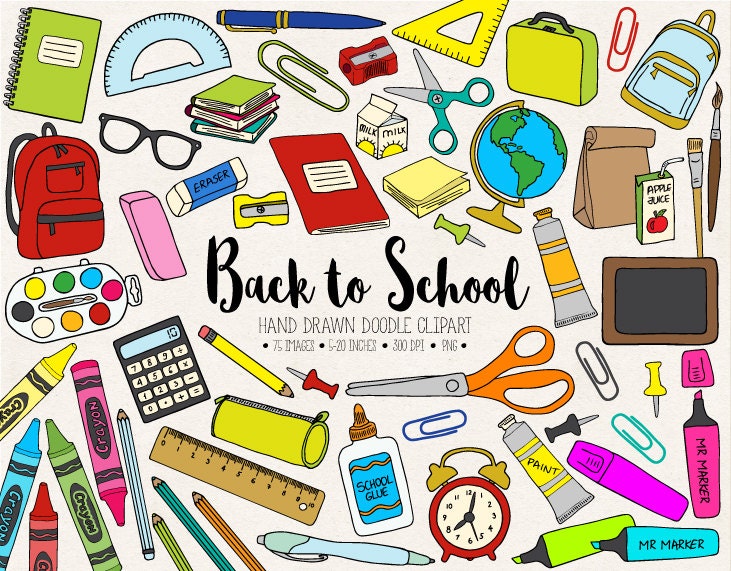This vibrant illustration, set against a white background, features an array of hand-drawn doodle clip art images centered around a "Back to School" theme. In the middle, bold black cursive text reads "Back to School," with smaller skinny text below stating "hand-drawn doodle clip art." Beneath this, a horizontal list details key features: "75 images, 5 to 20 inches, 300 DPI, PNG."

Surrounding the text are colorful and varied illustrations of school supplies, meticulously detailed to capture their essence. The assortment includes green notebooks, blue and yellow protractors, a green and yellow lunch box, a blue and brown backpack, and a range of writing implements such as pens, markers, crayons, and colored pencils. Additional items include a red alarm clock with yellow bells, a carton of milk, a carton of apple juice, scissors, erasers, a pencil sharpener, a globe, glasses, paper clips, thumbtacks, Post-it notes, paintbrushes, highlighters, a red book bag, and a calculator. This clip art collection embodies the lively and diverse array of supplies essential for the back-to-school season.